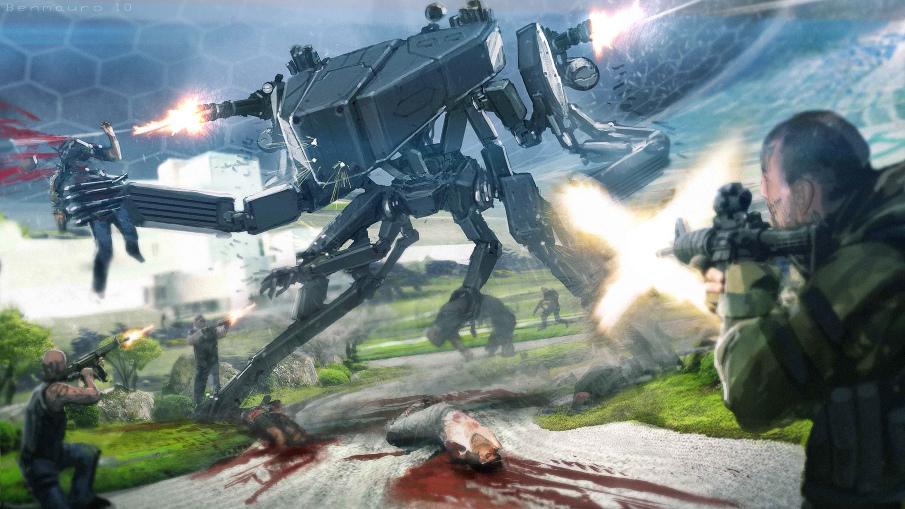In this detailed image, likely from a computer game, we see a huge, menacing robot dominating the scene. The robot, constructed from dark gray and silver metal, stands tall with a triangular head featuring two eyes and a mouth. Extending from various points on its body are six or seven arms, some of which are equipped with guns, including twin Gatling cannons on the top. In its right hand, the robot grasps a soldier, whose head has been gruesomely shot off. Another gun emerges from the back of its head, while a second protrudes over its left shoulder. The robot is depicted with two large, sturdy legs, one of which is firmly planted on the ground among several bloodied bodies of fallen soldiers.

Adding to the chaotic scene, the ground is littered with dead and injured soldiers, while others continue to fire their automatic rifles at the relentless machine. In the lower right corner, a man in a green uniform shoots at the robot, and in the left corner, another soldier kneels while firing. The battleground features a green landscape interspersed with paved areas, set against a striking sky with a honeycomb pattern. Above the battlefield, a large sphere with a hexagonal tiled surface adds a surreal element to the sky. The image captures a moment of intense combat and devastation as the soldiers strive to combat the overwhelming power of the robotic assailant.